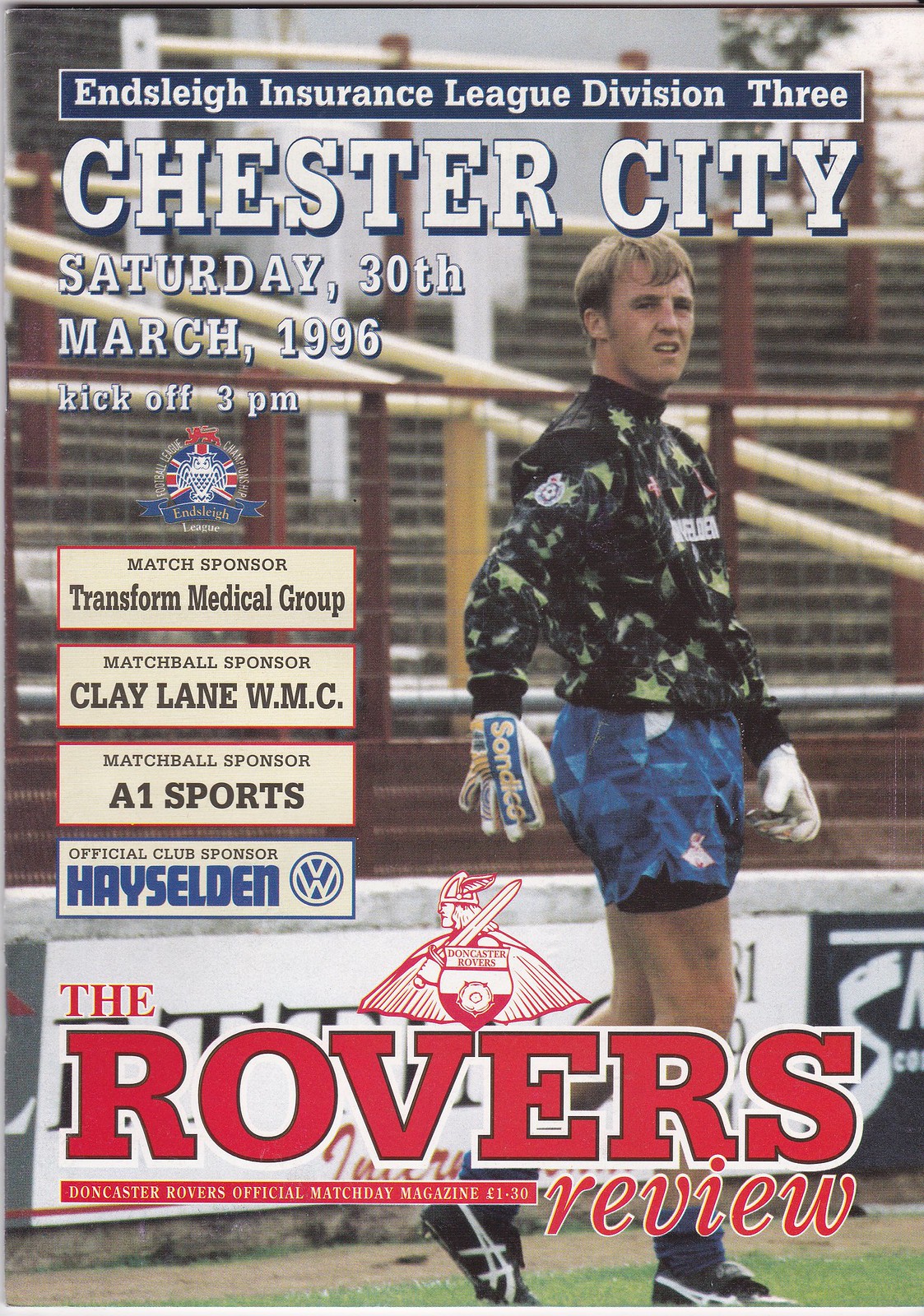The image appears to be the cover of a match day magazine for the Doncaster Rovers, titled "The Rovers Review," priced at £1.30. It prominently features text at the top reading "Enslay Insurance League Division 3 Chester City, Saturday 30th, March 1996, kickoff 3 p.m." in white letters on a blue background with a thin white border. Below this, it lists the sponsors: Transform Medical Group as the match sponsor, Clay Lane WMC and A1 Sports as the match ball sponsors, and Hayes-Seldon Volkswagen as the official club sponsor.

The central photo shows a soccer player standing on a grassy field, positioned in front of an empty spectator area. The player, possibly a goalie, is dressed in a distinctive outfit comprising blue shorts with black undershorts, and a long-sleeved black soccer jacket adorned with neon yellow stars and various designs. He also wears white gloves with the words "Sand Dust" inscribed on them and appears to be standing on some glasses. To the left of the image is a logo, while to the right is the tagline "The Rovers, Doncaster Rovers official match day magazine" in large red text.

In summary, the cover skillfully combines essential match details and sponsorship acknowledgments with a striking image of a goalie framed against the backdrop of an empty stadium, capturing the anticipation of the upcoming game.